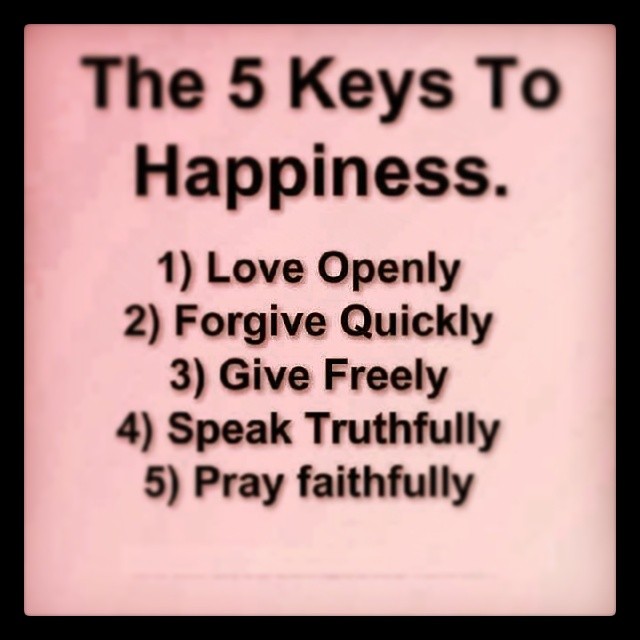The image is a square poster with a thin black border and a peachy pink background, reminiscent of the peach color from a colored pencil box. At the top, in bold black letters twice the size of the other text, is the heading "The Five Keys to Happiness." Below the heading, in smaller black letters, are the following five keys to happiness, each numbered with a small circle around the number: 1) Love openly, 2) Forgive quickly, 3) Give freely, 4) Speak truthfully, and 5) Pray faithfully. The simple yet impactful design makes it suitable for sharing on social media.